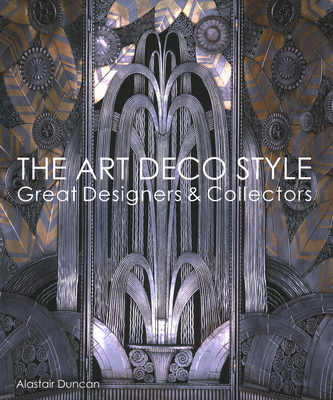In this image, there's a sophisticated Art Deco-style advertisement for a designer, prominently featuring the name Alistair Duncan at the bottom. The center panel is marked by an elegant display of metallic elements, mostly in shades of gray, silver, and black, with intricate light reflections creating a rich, bright appearance. This central area features a design reminiscent of water flowing from a fountain, with curved, looping stripes that arch and diverge in various directions. Flanking this centerpiece, the side panels display ornate patterns with gold and silver leaf-like motifs accompanied by round, flower-like designs. Across the whole image, white text reads "The Art Deco Style, Great Designers and Collectors," capturing the essence of the design and its aesthetic appeal. The overall palette includes tans and silvers, enhancing the luxurious metallic impression of the piece.